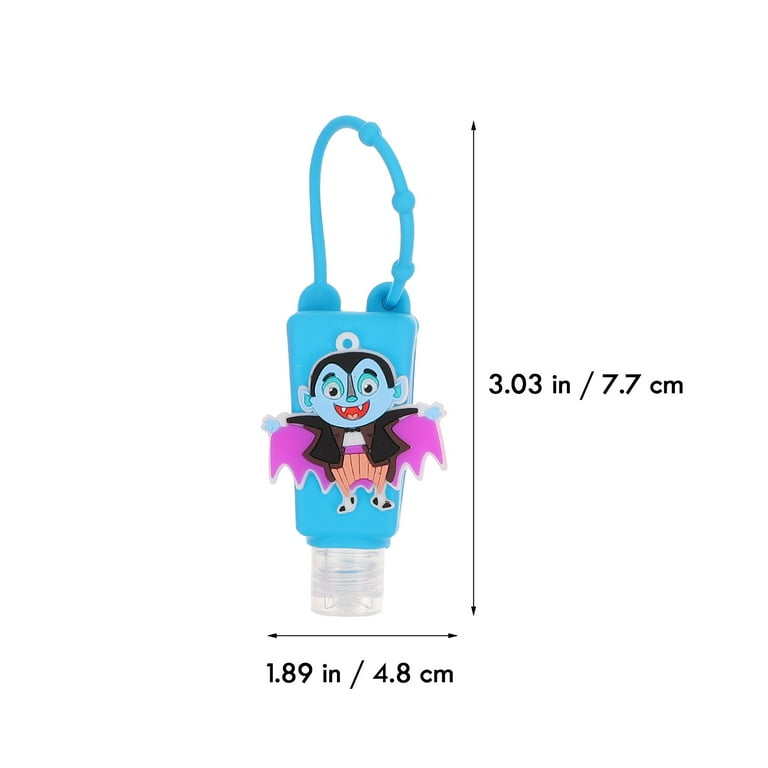This color photograph showcases a blue silicone hand sanitizer holder, designed with a vertical body that has diagonally tapered sides, allowing for a wider arc towards the top where a blue strap with circular blue beads is attached. The holder features a cutout of a cartoonish Count Dracula on the front, characterized by blue skin, black hair, googly eyes, a pink and black cape, and fangs protruding from a smiling red mouth. The height and width of the holder are labeled at the bottom of the image, measuring 3.03 inches (7.7 centimeters) in height and 1.89 inches (4.8 centimeters) in width. The blue strap enables the holder to be conveniently attached to various items such as a car interior or doorknob.